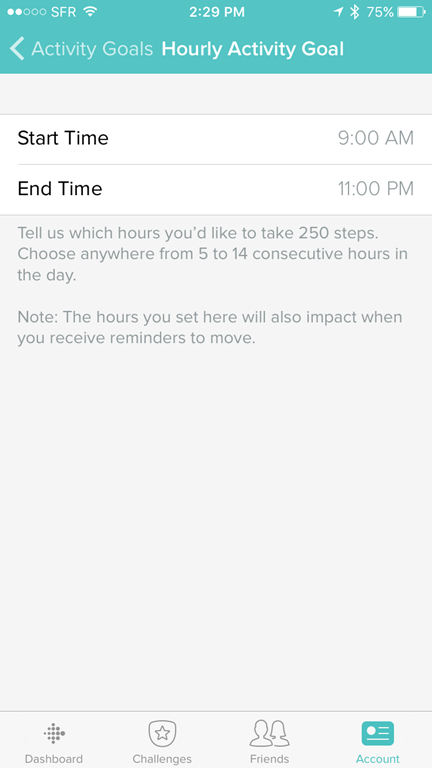The image displays a cell phone screen featuring a detailed and organized user interface. At the top, the status bar is colored teal. In the top left corner, there are five small circles with two filled in white. Next to these dots, the word "SFR" is displayed, indicating the mobile network. The Wi-Fi signal icon shows full strength.

Centered in the status bar, the time is displayed as "2:29 PM". To the right, there are icons for location services, Bluetooth connectivity, and a battery icon indicating 75% charge.

Below the status bar, the screen shows a section dedicated to "Hourly Activity Goals" with a back arrow on the left side. This is set against a gray background. Further down, there are fields for setting a start time and end time, listed as "Start Time: 9 AM" and "End Time: 11 PM", both in white sections.

Under these fields, there's another gray section with text that reads: "Tell us which hours you'd like to take 250 steps. Choose anywhere from 5 to 14 consecutive hours in the day. Note: The hours you set here will also impact when you receive reminders to move."

At the bottom of the screen are four icons representing different app sections. From left to right, these are: "Dashboard" (a diamond shape made up of dots), "Challenges" (a badge with a star in the middle), "Friends" (two silhouetted people), and "Account" (highlighted with a teal color).